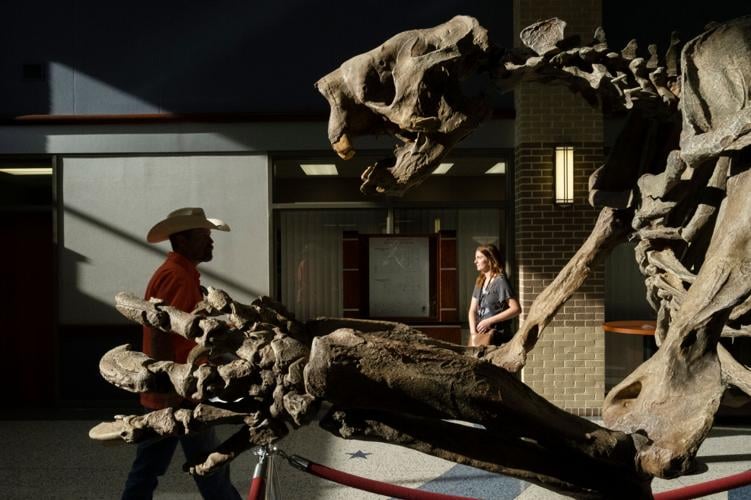In a dimly lit dinosaur exhibit at a museum, a towering, fossilized dinosaur with its massive, gray paw extended dominates the scene. The dinosaur's bones are a gray color, contrasting with its yellow or white-ish teeth. The exhibit is partially illuminated by fluorescent lights that run across the ceiling, casting shadows that enhance the room's dramatic ambiance. The exhibit background features white, blue, and gray walls, along with a gray projector screen and windows adorned with white blinds, framed by red bricks.

In the foreground, two individuals capture attention. A woman with dark brown hair, wearing a black or grayish shirt, leans against a brick pillar that has lighter gray on the bottom and darker gray on top. She is seen reaching into her brown purse. Nearby, an African-American man, dressed in a red shirt and a cowboy hat, stands in a position that makes it appear as though the dinosaur is interacting with him. The man sports blue jeans and moves closer to the exhibit, adding a touch of life to the still fossil display.

On the floor, the pattern alternates between blue and white tiles, and a distinct blue star is visible. A red rope barrier, attached to silver hooks, encircles the dinosaur to protect the exhibit. An additional element, a brown table with a black handle, rests in the background behind the dinosaur bones, adding to the intricate details of the room. The scene captures a moment of human fascination within a meticulously designed prehistoric display.